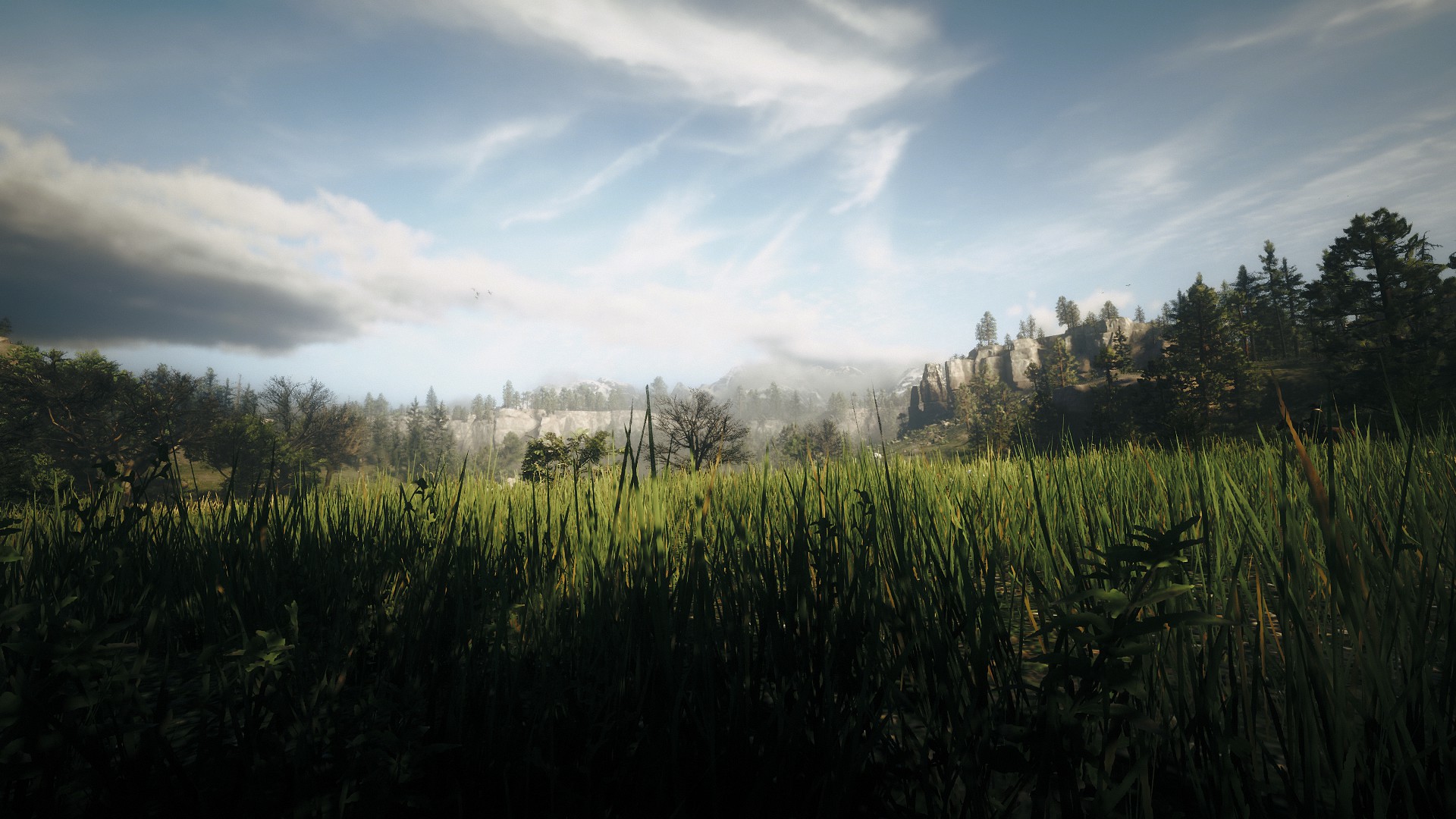The image depicts a highly realistic, possibly computer-generated or AI-created, scene of a grassy field. The viewpoint is low, almost as if the viewer is lying in the grass, with the top of the tall green blades dominating the foreground. The grass transitions from shadows at the bottom to bright, vibrant greens towards the top. In the distance, a dense array of trees, primarily pines and large leafy greens, lines the horizon alongside gray cliffs and potential mountains, partially obscured by clouds and what appears to be rain. The sky is a mix of soft blue and gray, filled with wispy clouds in various shades of white and gray, suggesting an impending storm. The overall composition showcases a striking contrast between the lush green foreground and the blue-gray sky, creating a vivid and immersive landscape.